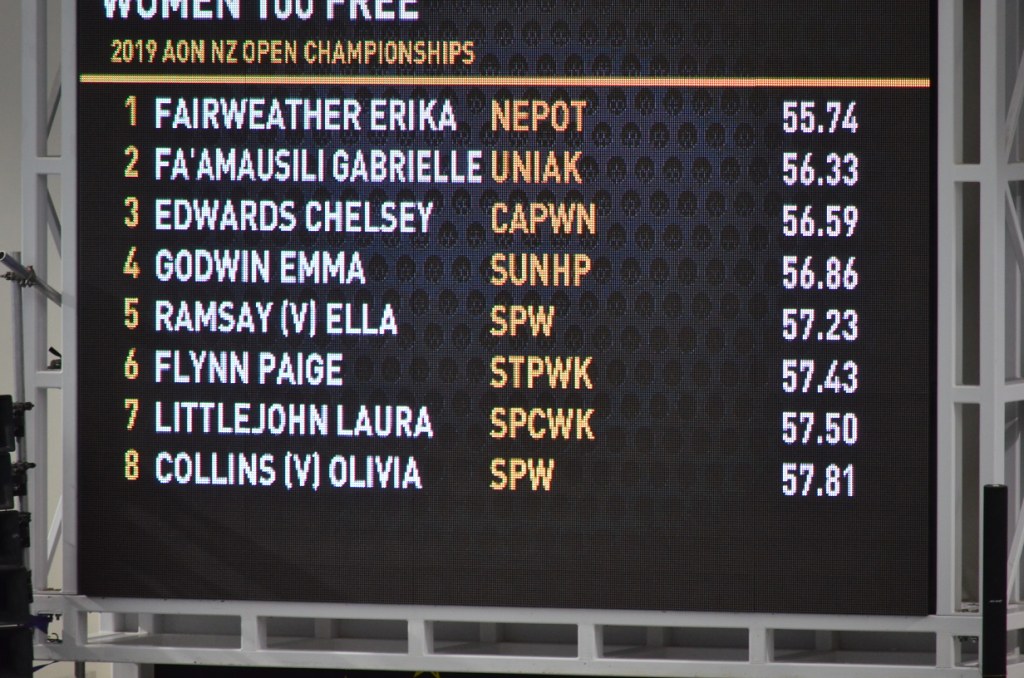The image depicts an electronic scoreboard with a black background and silver metallic frame. The top portion is slightly cut off but displays "Women 100 Free" indicating it's for the women's 100-meter freestyle event. Below this, in orange electronic lettering, is the title "2019 AON NZ Open Championship," suggesting it is a New Zealand championship. The scoreboard lists the top eight competitors:

1. **Fairweather Erica** - NAPOT, 55.74 seconds (white lettering for the name, orange for the location).
2. **Emmanuel Gabriel** - UNIAK, 56.33 seconds.
3. **Edwards Chelsea** - CAPWN, 56.59 seconds.
4. **Godwin Emma** - SUNHP, 56.86 seconds.
5. **Ramsey V Ella** - SPW, 57.23 seconds.
6. **Flynn Page** - STPWK, 57.43 seconds.
7. **Little John Laura** - SPCWK, 57.50 seconds.
8. **Collins V Olivia** - SPW, 57.81 seconds.

The entries are displayed in alternating white (for names and times) and orange (for locations) text across the black electronic screen.